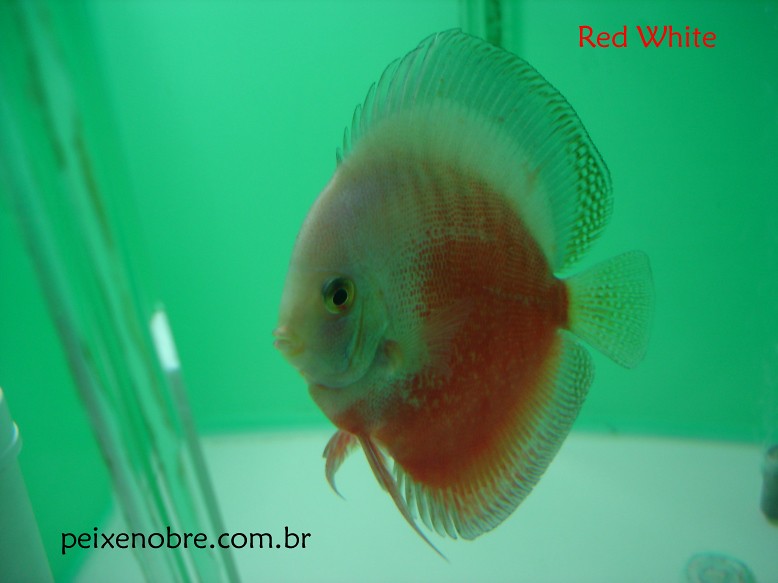This image captures a detailed scene inside a fish tank, framed by a slight view of the plastic or glass border on the left side. The tank appears to have a greenish hue, possibly from the background or lighting. Dominating the center of the image is a large fish, exquisitely detailed and positioned at a sideways angle. The fish, primarily featuring an orange body with a white face, has long, elegant fins on the top and bottom, and a small tail fin. Its fins are expansive, running nearly the entire length of its body. Surrounding colors in the image include green, tan, red, orange, black, yellow, and clear. In the top right, the text "RED WHITE" is prominently displayed in red, capital letters. Additionally, the bottom left corner features the website "peixenobre.com.br" in black text.